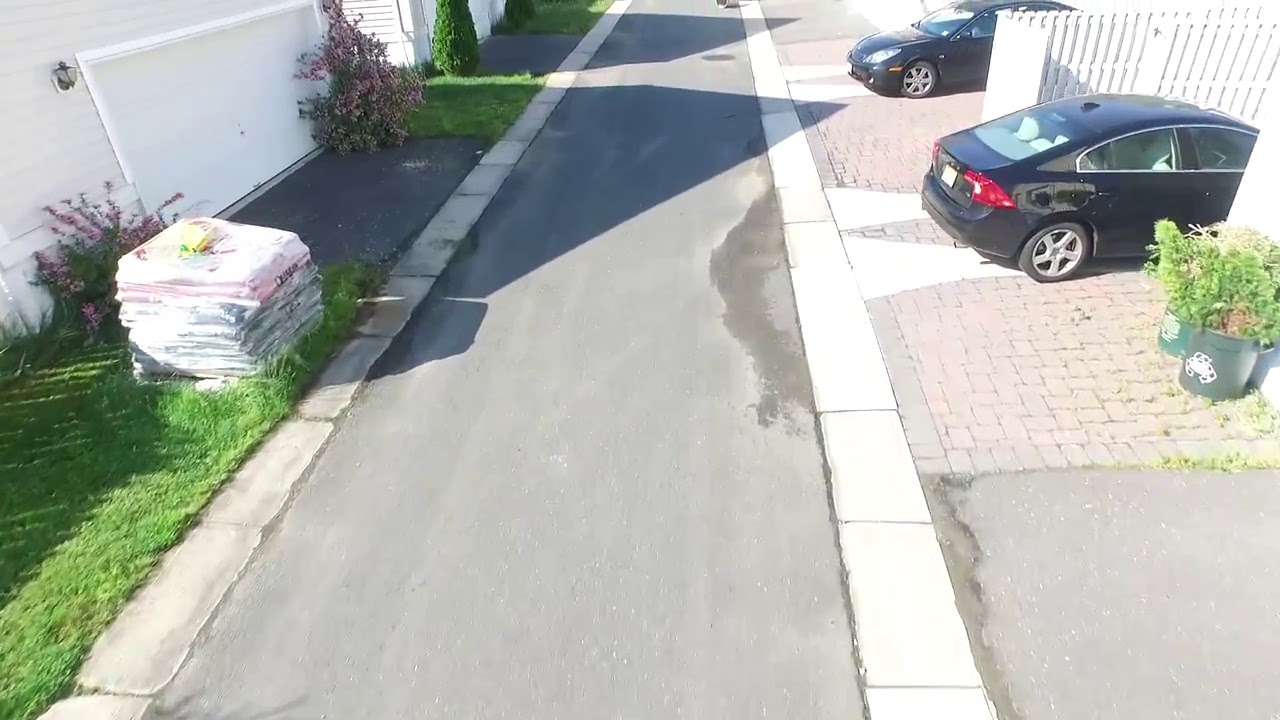The image appears to be taken from a high angle, possibly from the second story of a building, showcasing a narrow back road or alleyway typically found behind apartment complexes or homes. The road, which extends from the bottom to the top of the frame and is gray, accommodates barely enough space for two cars to pass. On the right side of the road, there are two black cars—one facing forward and the other facing backward—parked on brick-colored beige pavement. To the left, there are a couple of white garage doors connected to houses, alongside which is an area with green grass, plants, and what looks like a stack of large plastic-wrapped items. The stack consists mainly of white bags with the top two being pink, each about two feet wide, likely containing building materials. The overall setting suggests a sunny day in a quiet residential area.